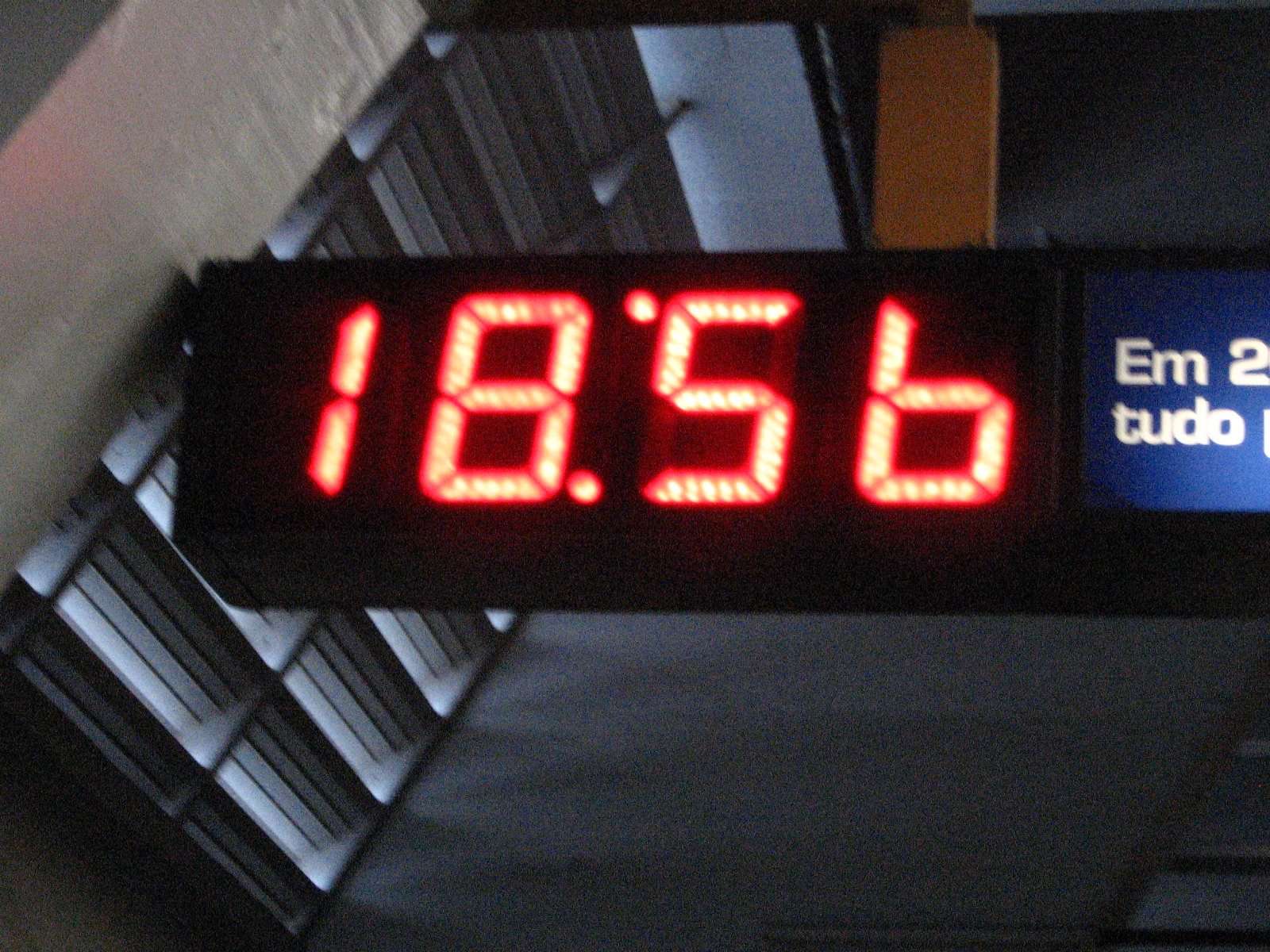This image seems to depict an antique clock or display piece hanging from a wooden structure. The clock, marked with the year 1856 in prominent red numerals, appears to be secured to a dark backdrop. To the right of the clock, partially visible text spells out "E M Tudor," although it’s somewhat obscured. The background shows a faint glow of light filtering through a grate or window, suggesting an older building or historical location. The wooden structure comes down from the top left corner, reinforcing the rustic and vintage atmosphere. The upper left portion of the image reveals part of the wall under natural light, adding depth and context to the scene.